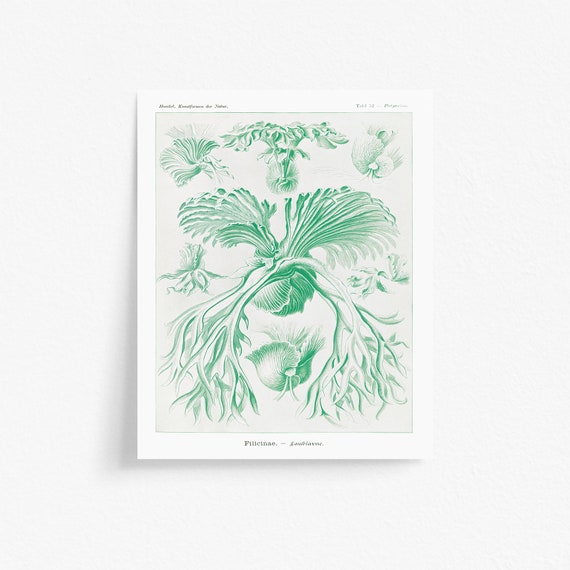The image depicts a beautifully detailed botanical illustration of green vines radiating from a central point, sprawling across a white piece of paper with a faint, lavenderish background. The vines extend gracefully in various directions, with the main branches arching dramatically down to the bottom left and right, while thinner, shorter tendrils stretch out to the top left and right. In the center of the composition, a prominent green bud emerges. The illustration is framed by a white, cardboard-like border, lending it a professional, almost scan-like quality. The word "Felicinae" is inscribed at the bottom of the image, indicating the plant family. Despite some blurred, gray lettering in the upper left corner, the central focus remains on the intricate, green foliage with delicate white accents throughout. Looking closely, one can see clusters of leaves and sprouting seeds, giving the appearance of a plant beginning to flourish.